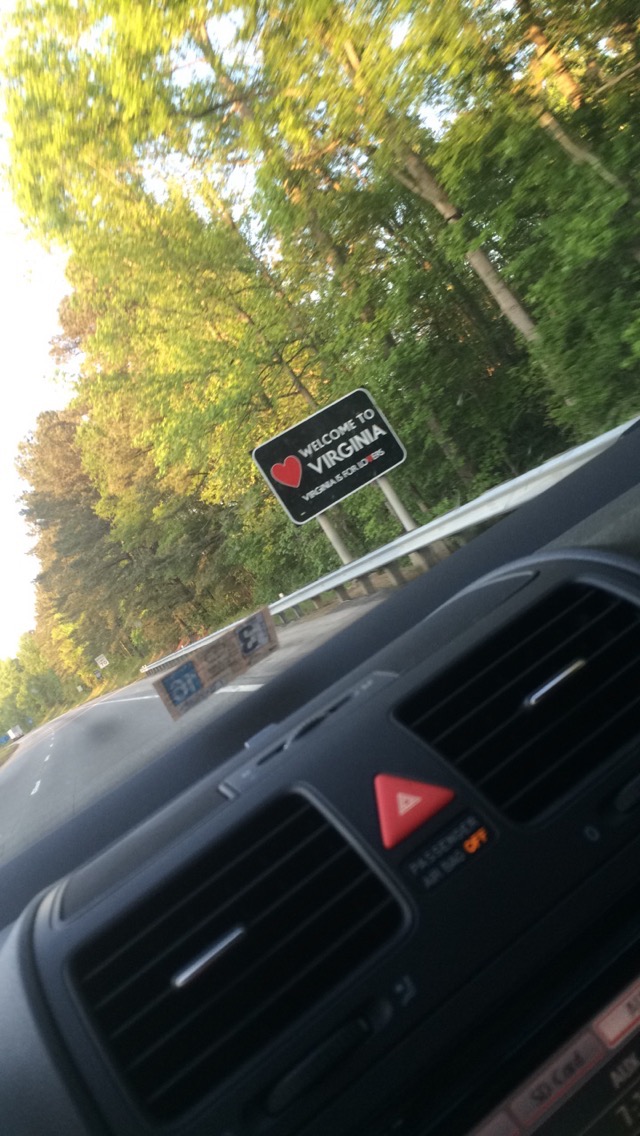The image, which is roughly two and a half times taller than it is wide, captures a scene from the front seat of a car with a black interior, specifically from the driver's perspective. Dominating the bottom half of the image is the dashboard, featuring two central air vents and a red hazard button between them, and an orange 'off' sign beneath it. Offset to the center of the image, you can see a registration sticker affixed to the windshield. The road ahead, illuminated by bright sunlight from the left, shows no immediate traffic, with a dotted line down the middle and a truck visible in the far distance. To the right of the road, behind a guardrail, stands a row of tall trees with green leaves resembling a forest. Centrally located on this side of the image is a black sign reading "Welcome to Virginia" in white text with a red heart to the left of the lettering. Additional text, partially obscured, is noted at the bottom of the sign. The top of the image is framed by the aforementioned row of trees, extending across the full width of the scene.